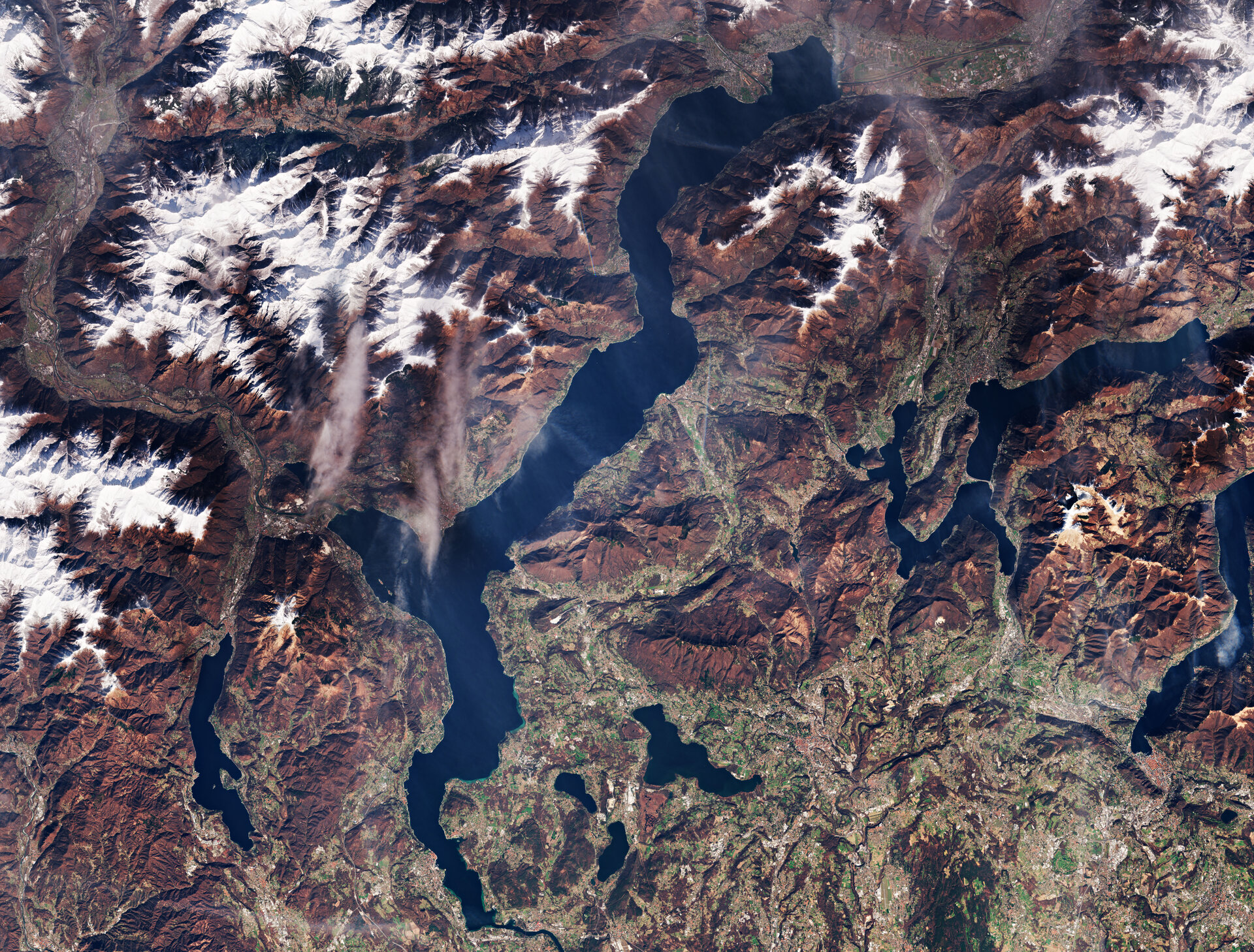This is an aerial or satellite photograph capturing a high-elevation, mountainous region with a mix of natural landscapes. The image shows a significant amount of water in the form of lakes and rivers snaking through the terrain, characterized by a dark blue color. Rising from the land are dark brown mountains, many of which have snow-capped peaks, indicating their high elevation. The lower elevations transition into lighter brown areas with patches of green, suggesting the presence of grass, trees, and other vegetation. The landscape is rugged and rocky, featuring exposed rock, with some regions covered in snow. There are wispy clouds partially obscuring parts of the view, but no man-made structures are visible, adding to the untouched, natural feel of this distant, elevated perspective of Earth.